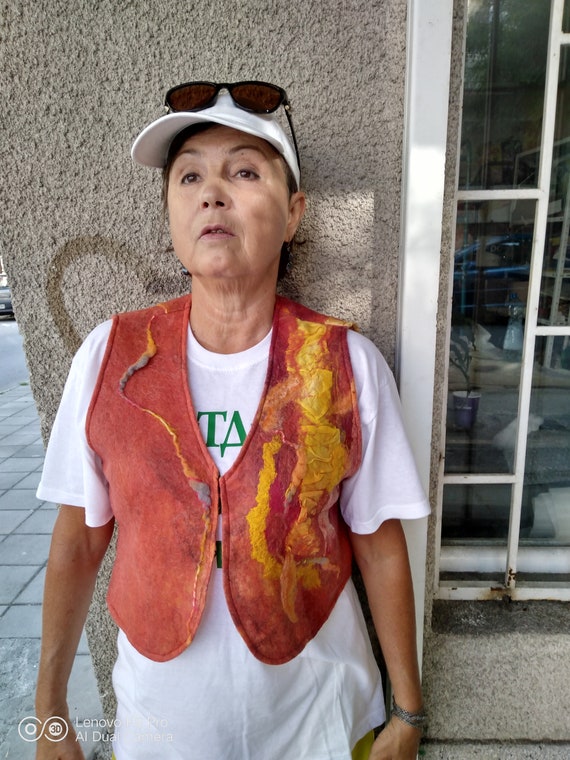In this full-color, vertically rectangular photograph taken outdoors in natural daylight, a middle-aged woman is standing with her back against a textured, gray stone wall of a building. She is wearing a distinctive, cropped red vest with yellow streaks that appear like paint patterns and a white t-shirt beneath, partially obscured but revealing the letters "T" and "A" across the front. The t-shirt features a green word, though it's mostly covered. The woman sports a white cap with sunglasses resting on top, and a bracelet adorns her wrist. She gazes straight ahead with a concerned expression, her arms hanging by her sides. To her right, a window reflects nearby buildings, a sidewalk, and a small plant in a planter. The scene is further detailed by a heart drawing on the brown stucco wall she leans against and a faint watermark at the bottom of the image.